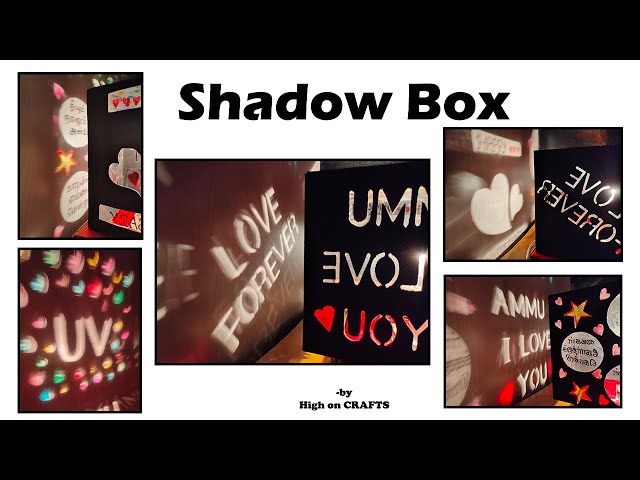This digital art display titled "Shadowbox," set against a white background with black bars at the top and bottom, features a series of intricate images. At the top center, "Shadowbox" is inscribed in bold black letters. The display includes five distinct images, arranged in a grid-like pattern. On the left, the topmost rectangular image showcases a complex mix of brown, black, and white colors with splashes of red, while the bottom rectangular image presents delicate pastel candy colors with the letters "UV" in pink and blurred hearts. The central, larger image is divided into two sections: the left with a brown background and the words "love forever" in white, and the right with a black background displaying an inverted reflection reading "U M" and "E V O L," followed by a red heart and "O Y U." Below this, in small black letters, it states "by High on Crafts." 

On the right side, at the top, another image mirrors the "love forever" text on a black background alongside a brown-toned image. The bottom right image features a brown section with "AMMU" and "I love you" in white letters, paired with a black section decorated with gray circles containing illegible text, pink hearts, and golden-orange stars. Overall, the display artistically mixes themes of love, utilizing light and shadow to convey various heartfelt messages.